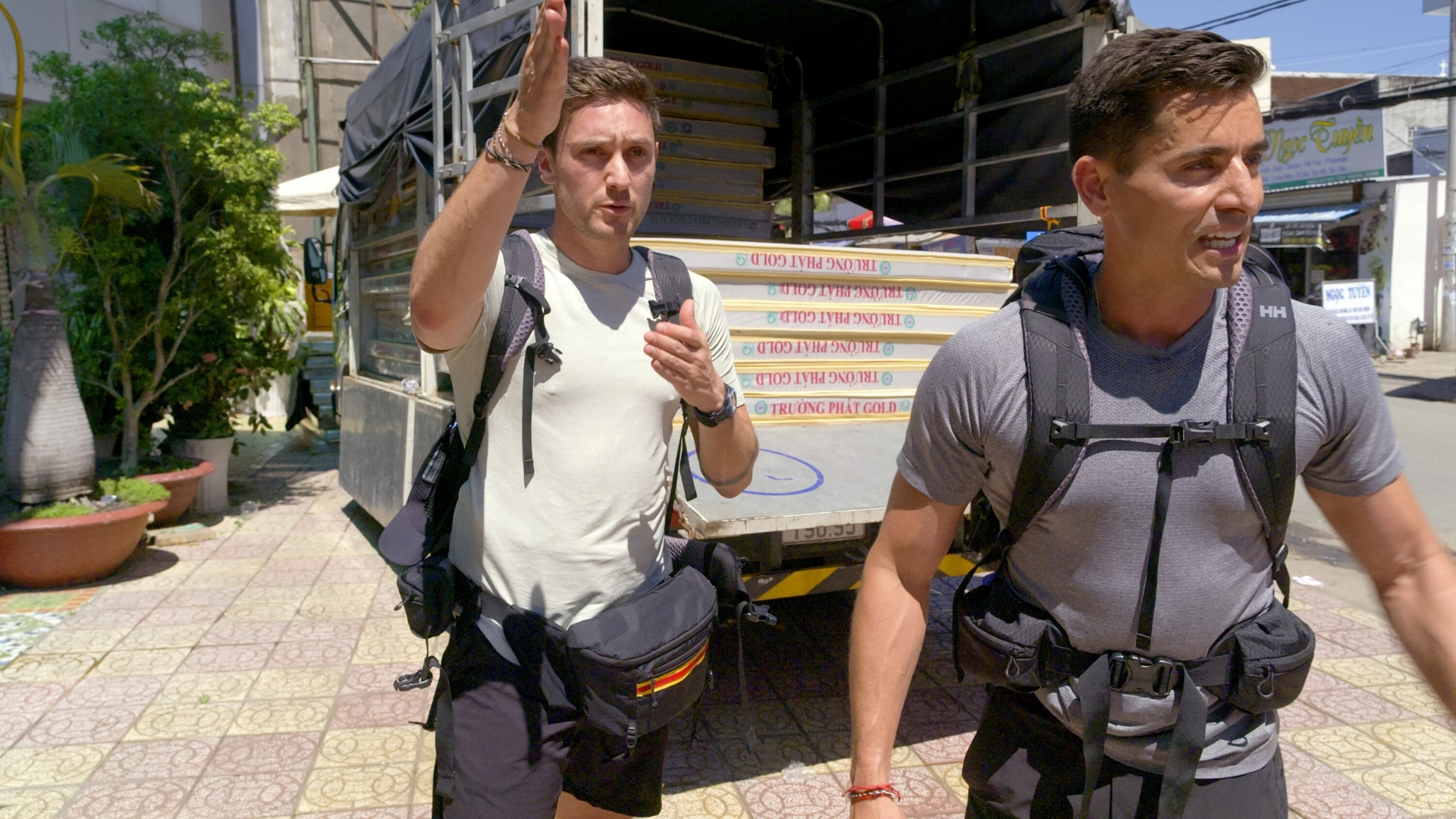In this vibrant daytime scene, two young men, potentially moving or delivery workers, stand outside near the open back of a trailer, which is filled with several identical boxes, possibly containing building materials. Positioned on a tiled walkway composed of yellow, pink, gray, and white tiles, the man on the left sports a white short-sleeved shirt, a black fanny pack, and a backpack; he's gesturing towards something off-camera with his right hand held flat. The man on the right wears a gray short-sleeved shirt and shorts, also equipped with a backpack and a waist pack, and looks to his left, seemingly preoccupied with something out of the frame. The background features a partial view of a building with an indiscernible blue sign, along with a mix of trees and orange planters, all under a clear blue sky indicating it's daytime. This scene likely captures a moment of coordination and communication amidst the bustling urban surroundings.